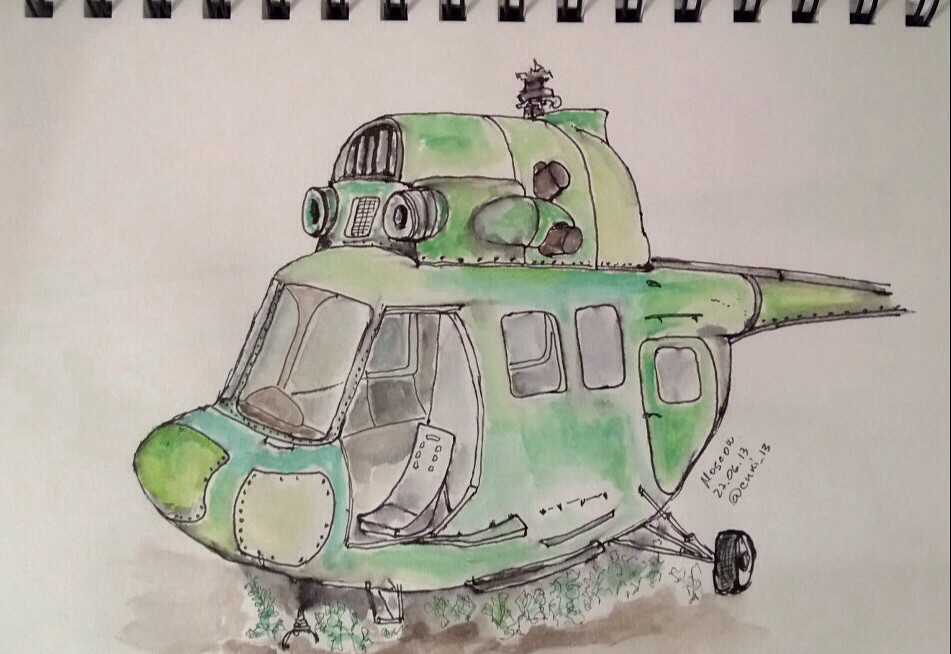The illustration depicts a green helicopter partially shaded with a technique resembling watercolors, on an off-white spiral notebook, evident from the visible spiral hooks at the top. The helicopter features a detailed body with an open door and a single seat for the pilot. The front windows are shown clearly, along with two side windows towards the back and a rear door. The landing gear is visible on the right side of the helicopter, including the small black wheel. The rear section of the helicopter extends out of the frame, leaving it partially cut off. Atop the helicopter's main body is a structure resembling a camera lens or pipes terminating in a circular end, accompanied by a black grill. This structure includes a small black tower and two minor black protrusions on either side. A patch of a different green shade and white marks are visible at the front of the helicopter. Underneath the helicopter, the artist has sketched tufts of grass, adding a touch of realism to the scene.